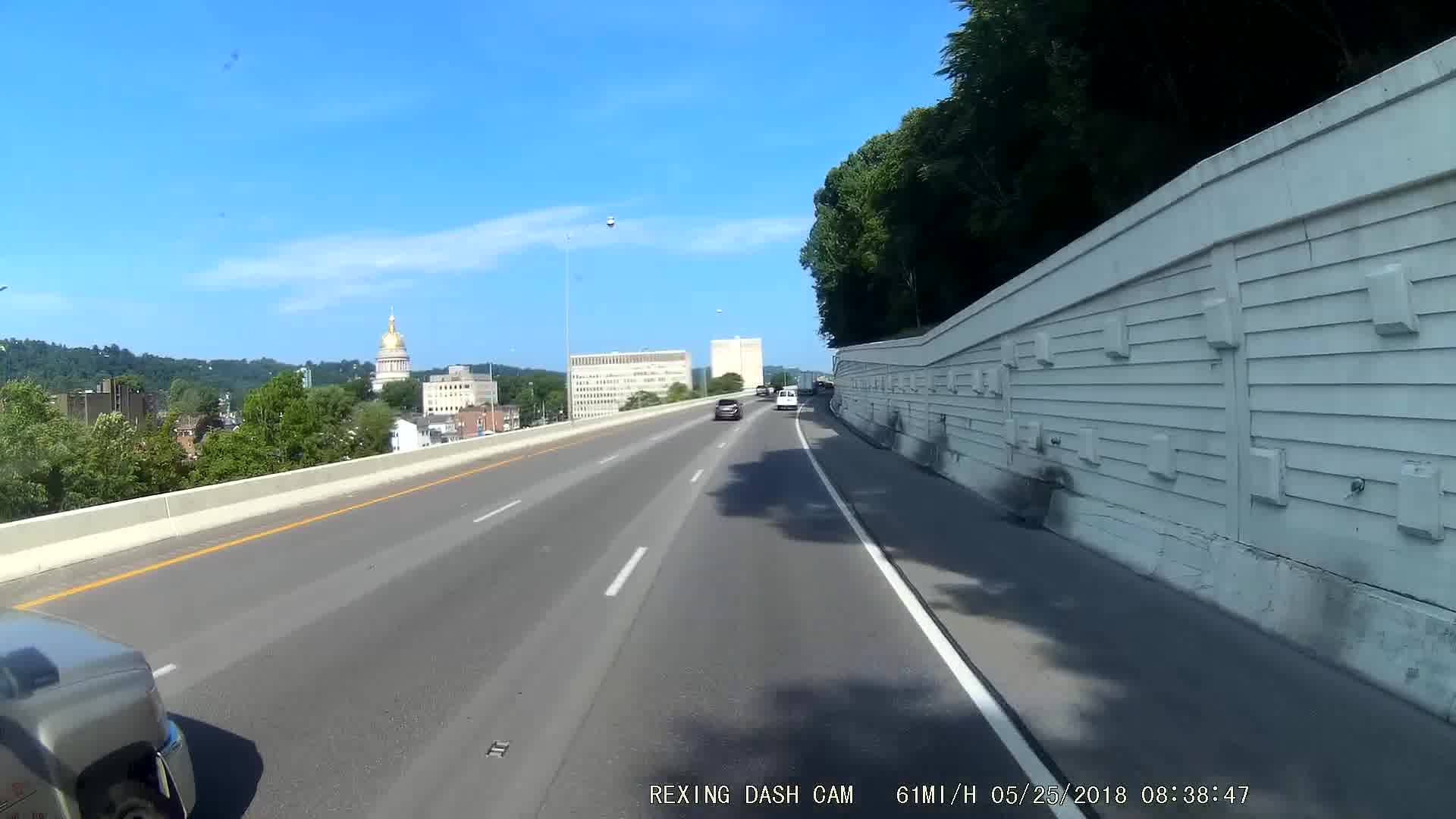The image shows a raised highway, with vehicles traveling in the same direction. On the right-hand side, a long white wall stretches alongside the road, with the tops of trees protruding above it. Three vehicles are visible in the distance, while a silvery grey car is just entering the foreground. A solid white line marks the right edge of the highway, indicating that this section may not be used for traffic, possibly serving as a lay-by or pedestrian pathway. To the left, more trees can be seen above the edge of the elevated roadway. In the background, white buildings are scattered among the trees, and a church is visible, adding a touch of architectural interest to the scene.